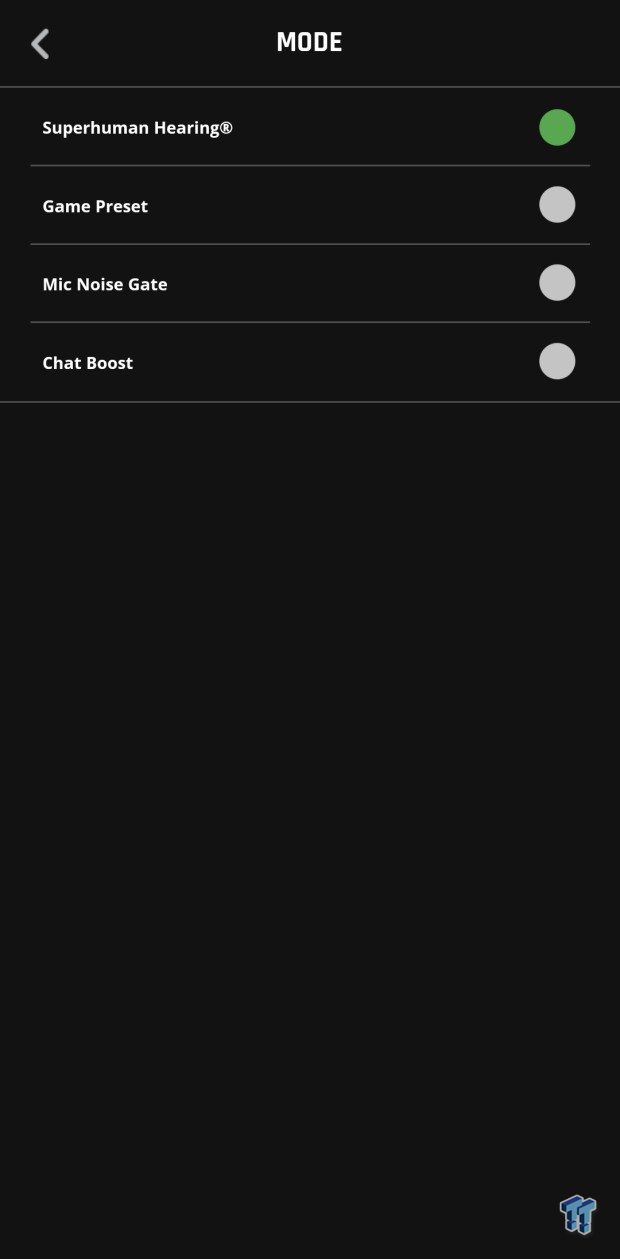This screenshot appears to be from an electronic device, though it's unclear whether it's a phone, tablet, computer, or another type of device. The screen itself is entirely black, with text and symbols displayed in white. At the top left corner, there is a back arrow symbol (<) indicating that pressing it would return the user to the previous page. Next to this arrow, the word "MODE" is displayed in all caps.

Below the header, there are four categories listed, each with associated buttons. The first category is labeled "Superhuman Hearing™," and it has a green button, which likely indicates that this mode is activated. The second category is "Game Preset," marked by a white button suggesting it's not active. The third category, "MIC Noise Gate," and the fourth category, "Chat Boost," also have white buttons next to them, indicating they are not active.

At the very bottom of the screen, there's a logo consisting of two Ts connected, depicted in blue against the black background. This symbol might be representative of the manufacturer's branding. The overall arrangement of the screen and the categorization implies that the interface could be related to audio settings, possibly for a gaming or audio-centric device such as headphones or a microphone.